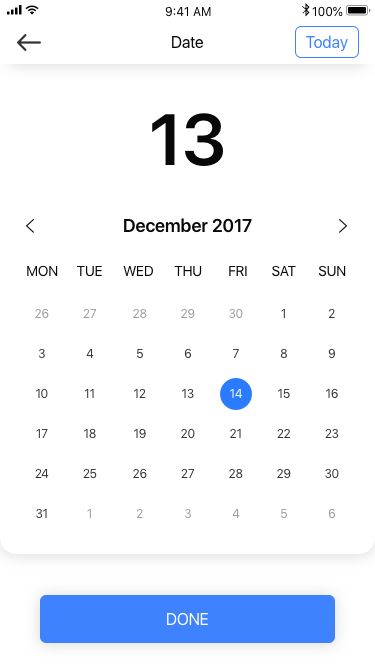The image showcases a calendar application displayed on a smartphone. At the top of the screen, the word "Date" is prominently shown in black, while the word "Today" is written in blue, situated at the top right corner. The main display indicates the calendar of December 2017, with the week starting on Monday and ending on Sunday. Notably, the 14th of December 2017, which falls on a Friday, is highlighted with a blue circle. The dates within the current month are written in black, whereas dates from the previous and following months are rendered in grey to provide clear differentiation. At the bottom of the screen, a blue button labeled "Done" in white text allows users to finalize their actions within the app. The overall background of the calendar interface is white, with black text indicating that the phone is in light mode. Additionally, there is a back button in the form of a left-facing arrow located in the top left corner for navigation to the previous screen.